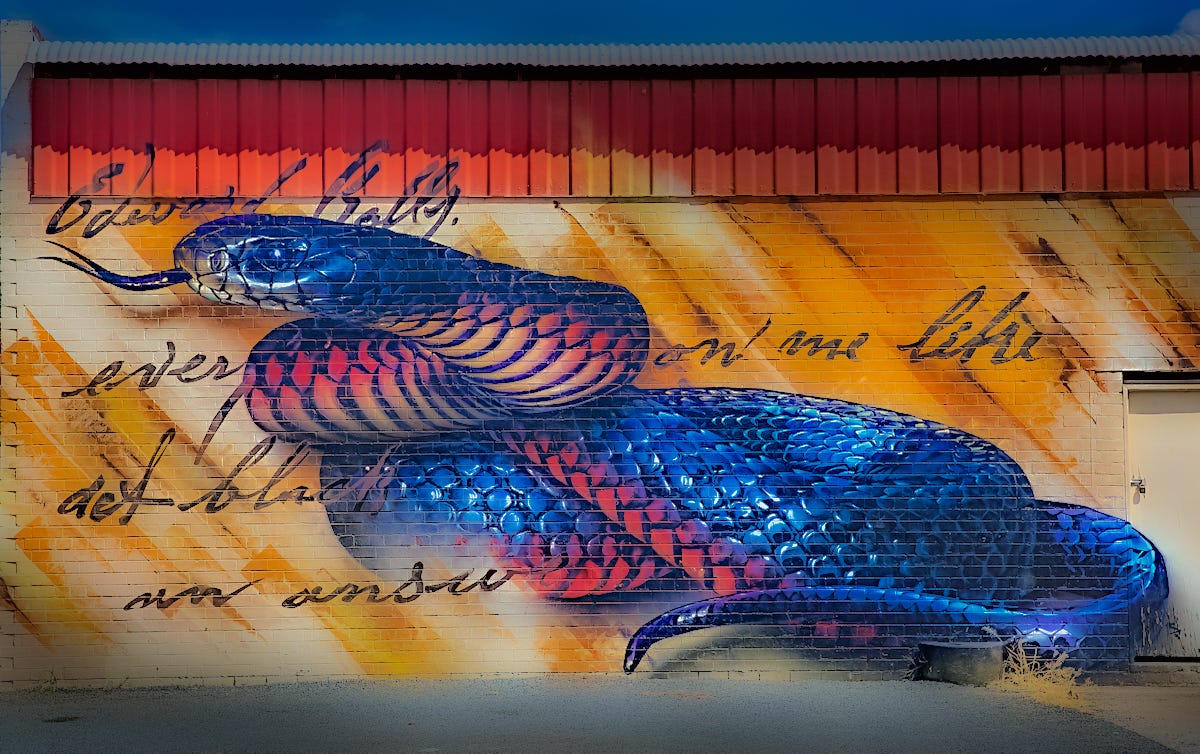The photograph depicts the side of a building adorned with a vibrant and professionally painted mural. The mural features a striking, coiled blue rattlesnake with a vivid cobalt blue back, a white underbelly, and a reddish hue connecting the two. The snake's scales shimmer as if painted with a gradient to imitate a natural sheen, and it extends a black tongue, contributing to its lifelike appearance. Surrounding the snake are words written in cursive, though not all of them are entirely legible, phrases like "ever on me like" and "deaf black" can faintly be discerned. The background of the mural is a dynamic montage of yellow, burnt orange, and brown hues, resembling crepuscular rays that streak diagonally across the brick wall. Additionally, there is a white door on the right-hand side of the building’s facade, and the top of the building features red shingles, adding to the overall picturesque scene.